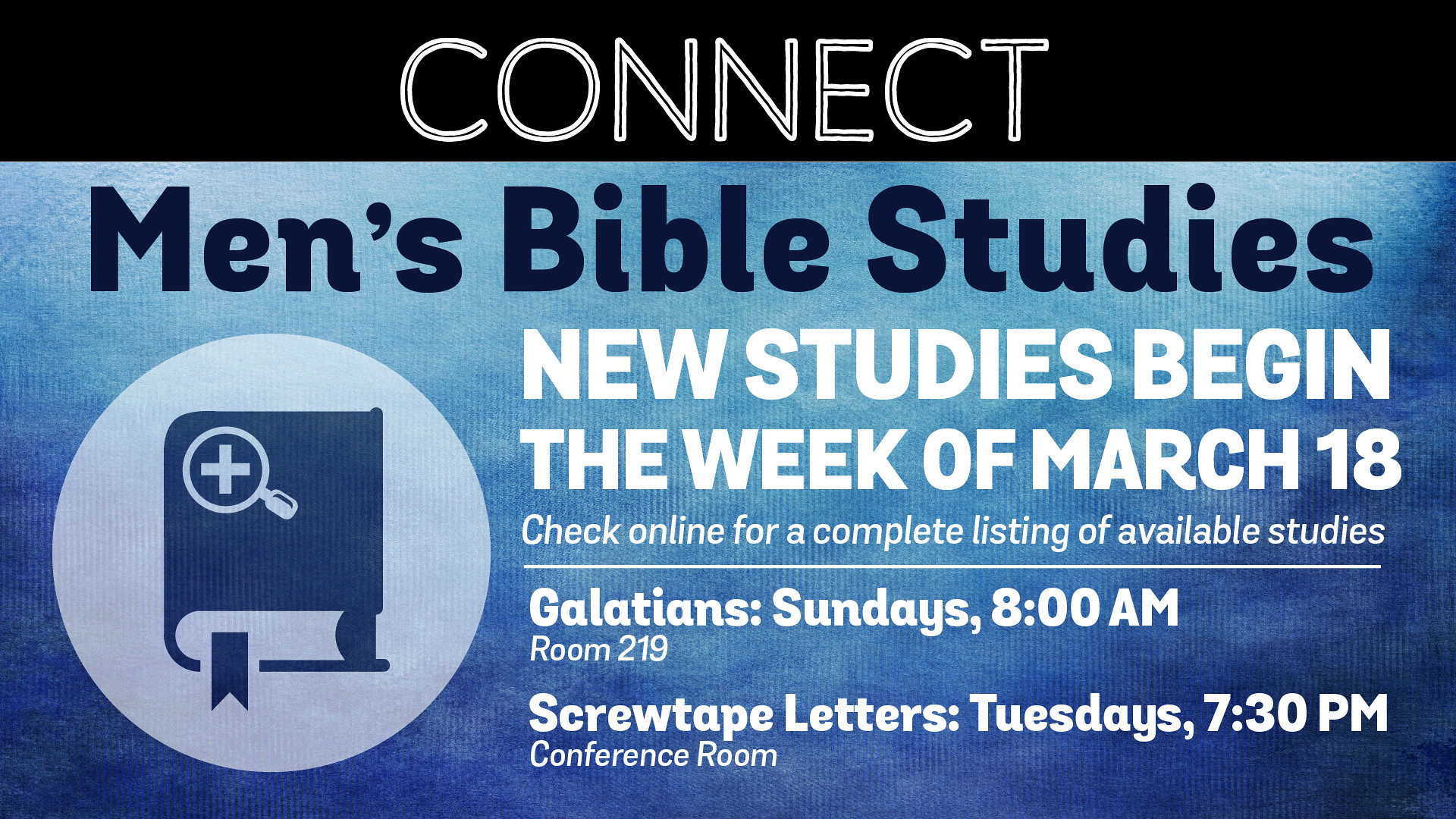This image appears to be an advertisement for men's Bible studies. It features a black header at the top with the word "CONNECT" in bold, white, capital letters. Below this, the text reads "Men's Bible Studies" in white, set against a black background. Important details about the studies are provided, highlighting that new studies begin the week of March 18th, with a prompt to check online for a complete listing of available studies. The advertisement further specifies two studies: "Galatians" on Sundays at 8 a.m. in room 219, and "Screwtape Letters" on Tuesdays at 7:30 p.m. in the conference room on the left. Additionally, there's a logo featuring a Bible with a bookmark and a magnifying glass with a plus sign on the top left corner of the book.